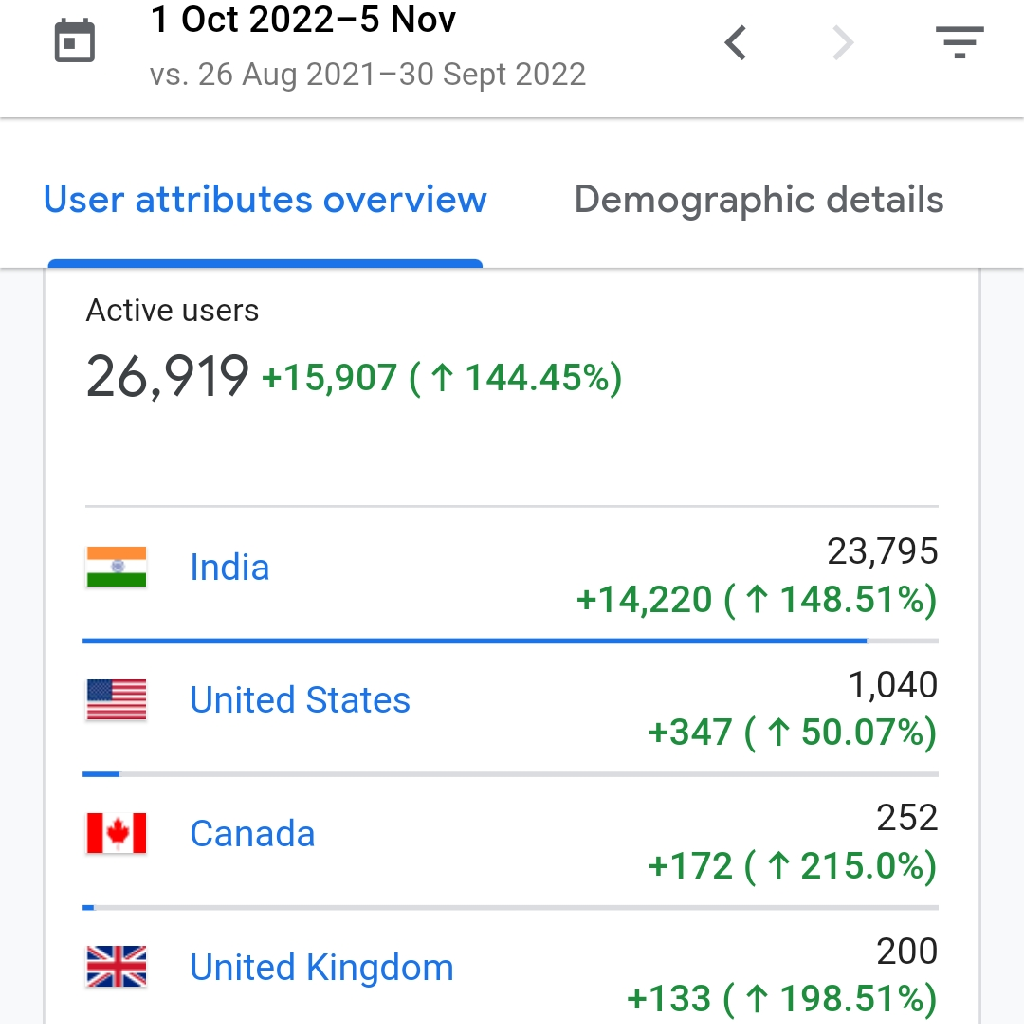A detailed caption for the described image could be:

"On a mobile site interface, a calendar at the top displays the date range from January 12, 2022, to November 5, 2022. Below, there are two tabs: 'User Attributes Overview' and 'Demographic Details', with 'User Attributes Overview' highlighted. This section indicates an impressive increase in active users, totaling 26,919, which is an increase of 15,907 users or a growth rate of 144.45% over the selected time period, slightly over a month. The geographical distribution of users shows a significant majority from India, accounting for over 23,000 users. Other notable user counts include approximately 1,000 from the United States, 250 from Canada, and 200 from the United Kingdom. The exact nature of the app remains unspecified, but it is focused on tracking and displaying user growth and demographic distribution."